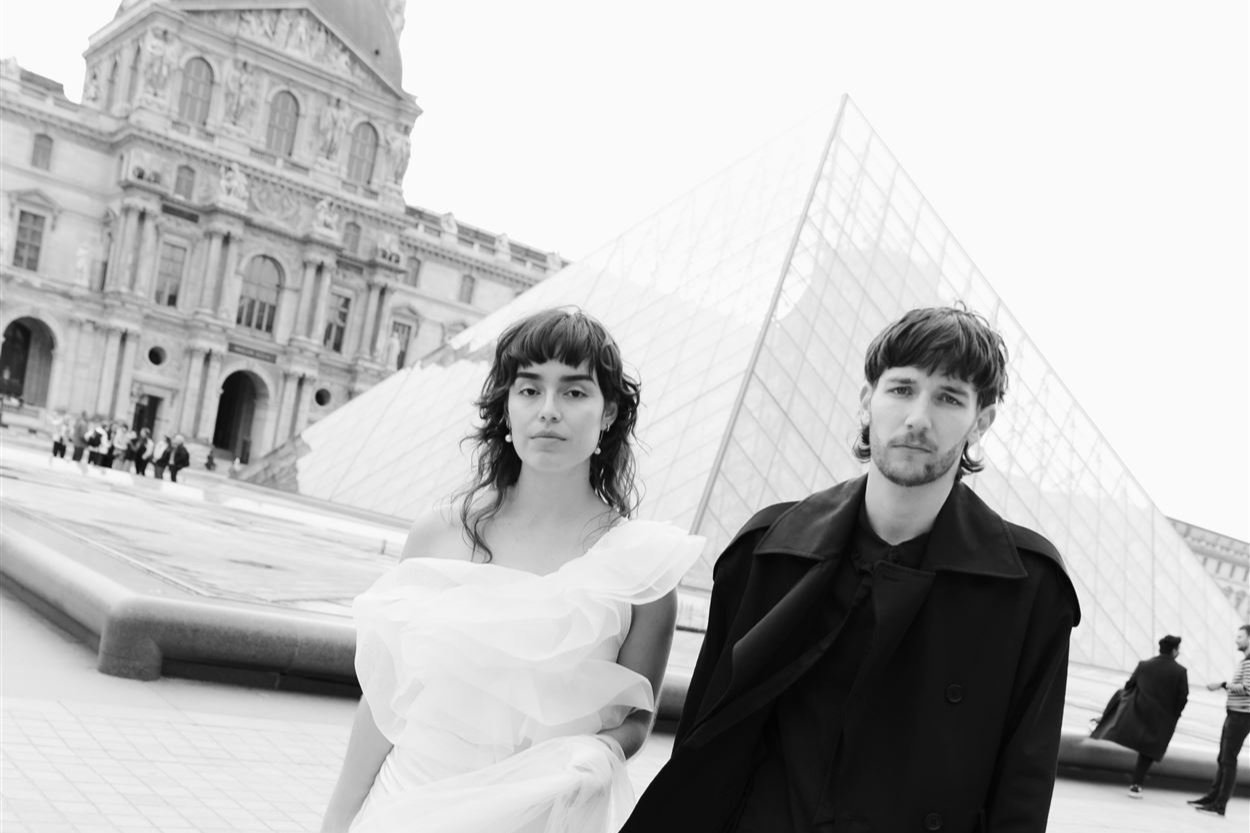In this black-and-white photograph, a stylish couple in their mid-twenties stands in front of the iconic glass pyramid of the Louvre Museum in Paris. The man on the right has black hair, a slight beard, and is dressed in a black jacket and shirt, while the woman on the left wears a one-shouldered, frilly white dress that leaves her right shoulder bare. Her medium-length black hair cascades down, complemented by white earrings. The dress resembles wedding attire but isn't quite as elaborate. Both wear serious expressions as they gaze directly into the camera. The image, shot from a diagonal angle, includes the grand, ornate Louvre building with its arched windows and statues in the background. The scene also reveals glimpses of a few people near the sculpture behind them and scattered further into the distance, reflecting a serene yet captivating moment frozen in time.